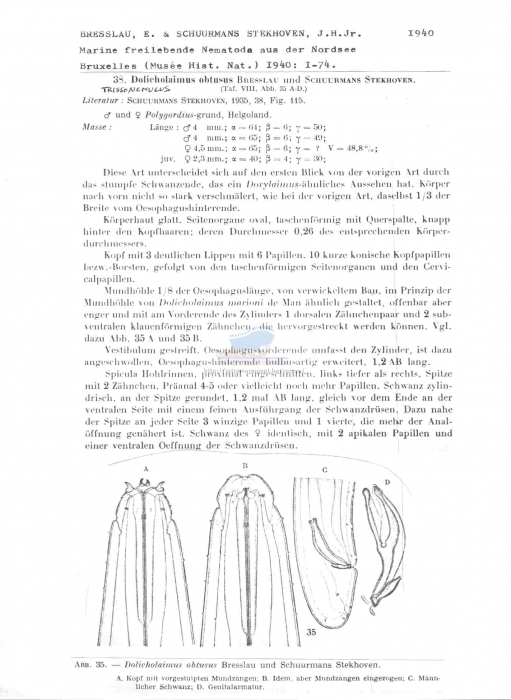The image is a scanned page from a dense, text-heavy textbook, possibly written in German and likely from a 1940 publication, as indicated by the number stamped in the upper right corner. The top of the page features formula equations and complex symbols, followed by six lengthy paragraphs of dense black text, rendering it unreadable without knowledge of the language. The content suggests an academic or scientific nature, possibly related to marine biology or entomology. The lower third of the page displays four diagrams labeled A through D, depicting creatures that resemble insects or aquatic organisms. Further details include footnotes at the bottom of the page and a white background with black text throughout.